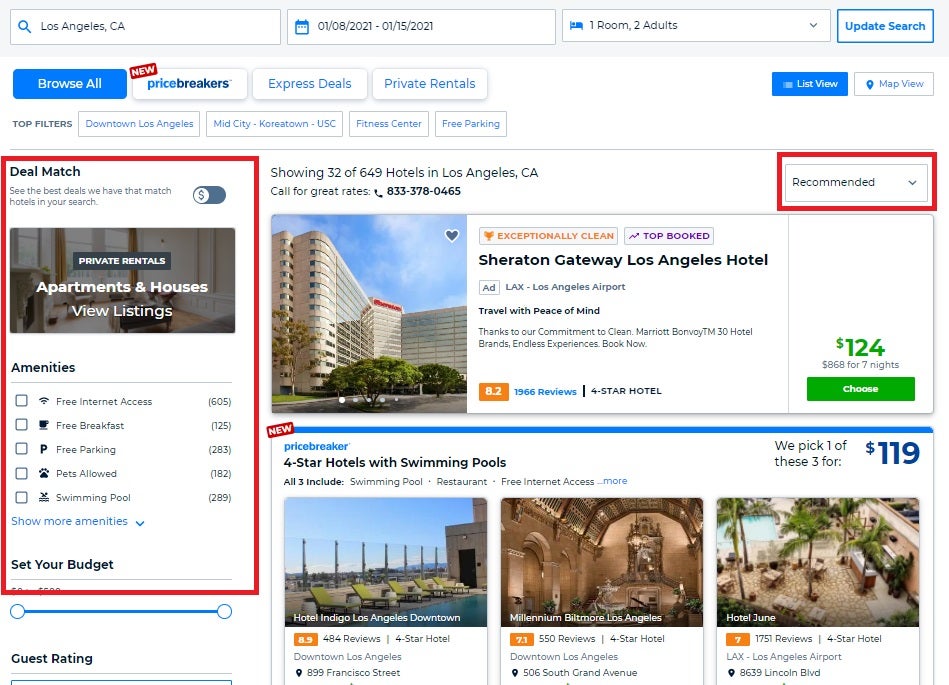Explore a plethora of hotel options in Los Angeles, California on this user-friendly travel website. Navigate easily with the search box located at the top of the page, where you can input your desired location, arrival and departure dates, number of guests, and rooms needed, before clicking the 'Update Search' button. Fine-tune your search results through various filters such as 'Browse All,' 'Price Breakers,' 'Express Deals,' and 'Private Rentals.'

Beneath these options, refine your search using 'Top Filters' such as Downtown Los Angeles, Mid-City, Koreatown, USC, Fitness Center, and Free Parking. Specific amenities like free internet access, free breakfast, free parking, pet-friendly accommodations, and swimming pools are highlighted in red boxes under the 'Deal Match' filter to further narrow down your preferences.

On the right side of the page, a filtered section allows you to sort hotels by different criteria with a dropdown menu currently set to 'Recommended.' Featured prominently is the Sheraton Gateway Los Angeles Hotel, priced at $124 a night. The listing includes a compelling visual of the hotel, an enticing 'Choose' button in green, and a high rating of 8.2, making your decision-making process seamless and informed.